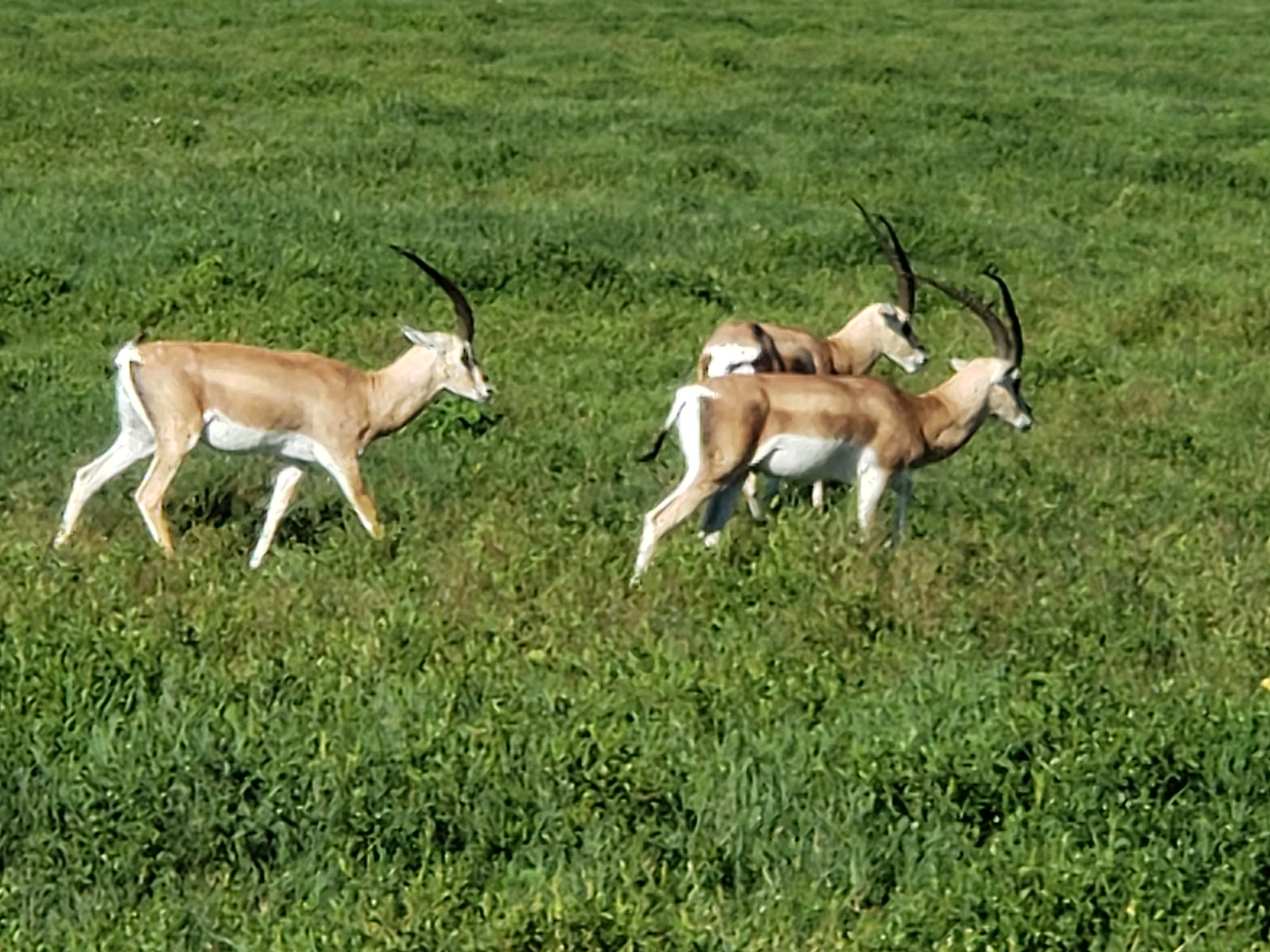The image features three antelope-like animals with distinguishing large, black, backward-curving horns. Their bodies exhibit a light brown color on the upper parts, transitioning to white on their underbellies, inner legs, and tails. They are set in a dense, lush field of predominantly green grass with some light brown patches, possibly due to flowers or variations in the grass. All three animals face towards the right side of the frame, with the two in the front aligned closely, and the third positioned slightly behind and at a different angle, appearing to turn. The photograph is taken outdoors under a sunlit sky, with the expansive field stretching out in every direction, indicating a natural, untamed environment rather than a controlled setting like a zoo. These creatures move leisurely, seemingly at ease, as they navigate the tall grass with long strides, creating an impression of serene coexistence with their habitat.